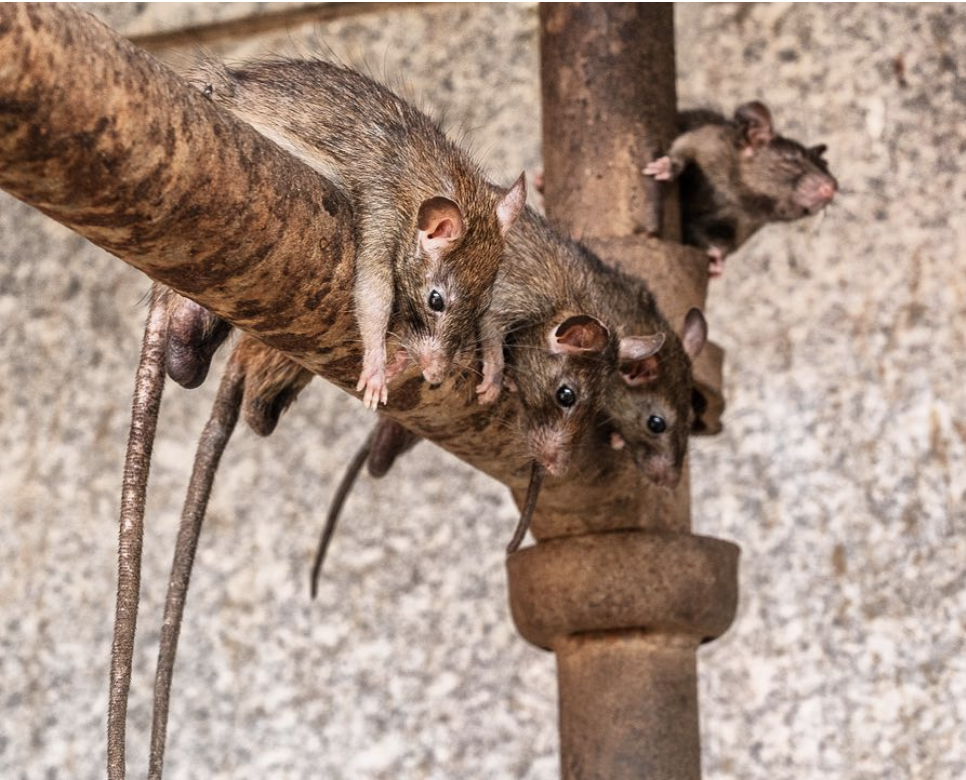The image captures four brown rats perched on a rusty T-shaped pipe, which contrasts starkly against a speckled rock wall backdrop in shades of white, gray, and brown. Three of these rats are stretched out across the horizontal section of the pipe, their bellies pressed against the rusted metal and their tails dangling behind them. They appear to be engrossed in observing something on the ground below, their little bodies and long tails extending towards the viewer. Meanwhile, the fourth rat, situated on the vertical section of the pipe, peeks around the corner, its crinkled nose and eyes suggesting it's sniffing the air, perhaps eavesdropping on this little rat gathering. The entire composition, framed within a rectangular six by five-inch photograph, evokes a scene of casual curiosity amidst a backdrop of aged industrial elements.